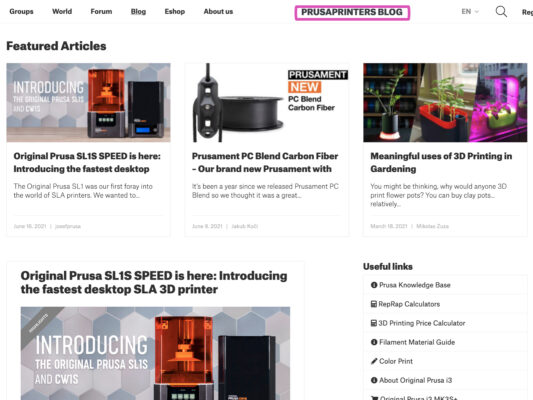**Detailed Caption:**

The image is a detailed screenshot of a website related to 3D printing, focusing on the "Original Prusa SL1SB" 3D printer. 

In the top left corner of the screen, there are navigation links labeled "Groups," "World," "Forum," "Blog," "eShop," and "About Us." Below these, a purple rectangle displays the title "Printer's Blog," followed by the names "Ian," "Amanda," and "Megan."

A prominent section titled "Feature Articles" appears to list various topics, with one particularly highlighted section introducing the "Original Prusa SL1SB." The section includes text that describes a 3D printer encased in an orange plastic shell with a hex-shaped back. The text suggests that this model is a new release from Prusa, following the success of their previous models like "Prusa Man" and "PC Blind." The caption emphasizes that the Prusa SL1SB is fast, accessible, and useful for practical applications of 3D printing.

Additionally, the image includes close-ups of the 3D printer's plastic casing and directs visitors to useful resources such as the "Prusa Knowledge Base," "Carify Calculators," "3D Printing Price Calculator," the "Filament Material Guide," and color printing information.

The bottom section of the image contains dense text about the "Original Prusa SL1SB," offering detailed insights into its features and practical uses in the field of 3D printing.